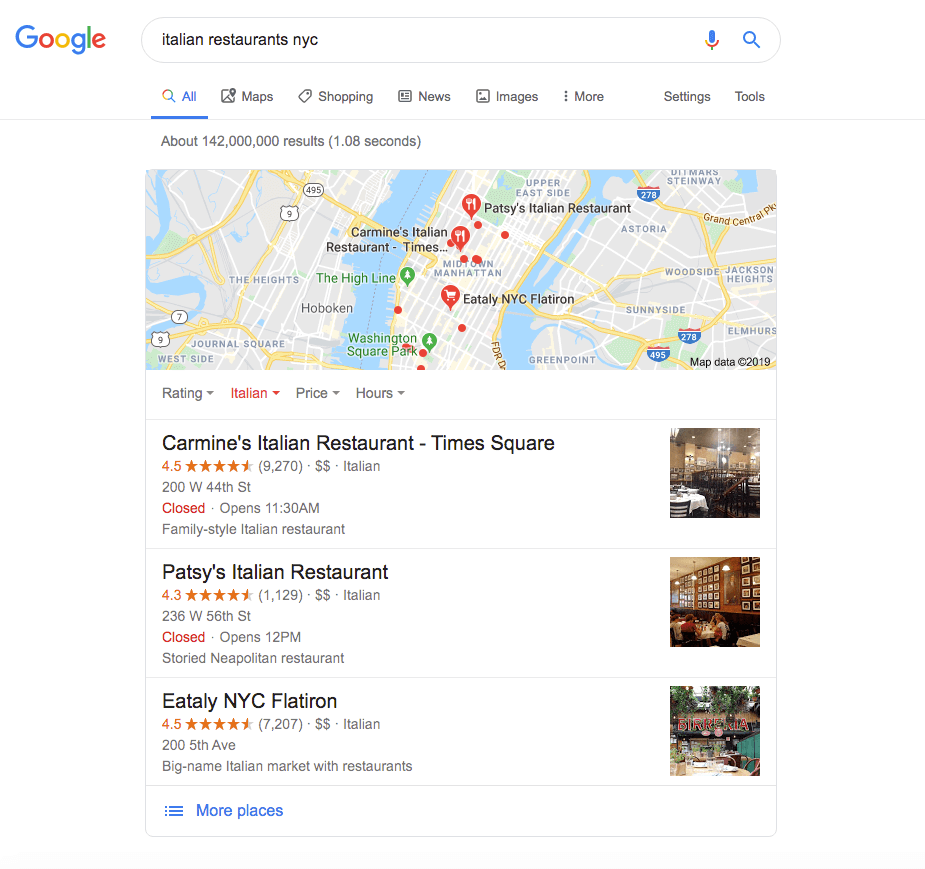The image is a screenshot of a Google search results page. At the top left corner, the iconic Google logo is visible, displaying the letters in a colorful combination of blue, red, yellow, blue, green, and red. In the search bar, the query "Italian restaurants NYC" is entered, accompanied by a microphone icon and a magnifying glass icon on the far right.

Below the search bar, there is a menu bar featuring various options: "All" (which is currently selected), "Maps," "Shopping," "News," "Images," "More," "Settings," and "Tools." The search has yielded approximately 142 million results in just 1.08 seconds.

A map of Midtown Manhattan is prominently displayed, with several marked locations indicating the Italian restaurants in the area. Notable entries include Patsy's Italian Restaurant, Carmine's Italian Restaurant, Times Square, and Eataly NYC Flatiron.

Below the map, three vertical photographs showcase different Italian restaurants, along with detailed descriptions:
1. **Carmine's Italian Restaurant, Times Square**: Rated 4.5 stars out of 9,270 reviews, denoted with two dollar signs ($$) suggesting moderate pricing. Located at 200 West 44th Street, the restaurant is closed at the moment and will open at 11:30 a.m. It is described as a "Family Style Italian Restaurant."
2. **Patsy's Italian Restaurant**: This establishment has a 4.3-star average from 1,129 ratings, also marked with two dollar signs ($$). It is located at 236 West 56th Street and is currently closed, set to open at 12 p.m. Patsy's is known as a "Storied Neapolitan Restaurant."
3. **Eataly NYC Flatiron**: Featuring a 4.5-star average rating from 7,207 reviews, and denoted with two dollar signs ($$). It is situated at 200 Fifth Avenue. Eataly is described as a "Big name Italian market with restaurants."

At the bottom of the page, a "More Places" link invites users to explore additional dining options.